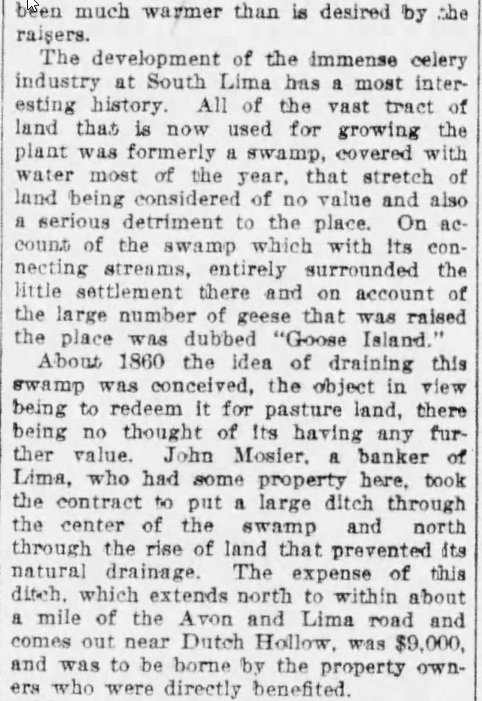This image is a clipping from a newspaper article discussing the intriguing history of the celery industry in South Lima. The article highlights how the vast tract of land now used for growing celery was once a largely water-covered swamp, deemed a significant detriment to the area and of no practical use. This land, which was surrounded by connecting streams and home to many geese, was historically known as Goose Island. Around the year 1860, an initiative to drain the swamp was undertaken with the intention of converting it into pastureland, without an initial expectation of any further value. John Mosler, a banker from Lima who owned property in the area, spearheaded the project. He contracted to construct a large ditch through the center of the swamp, allowing for proper drainage. This ditch extended north to about a mile from the Avon and Lima Road and emerged near Dutch Hollow, costing $9,000, an expense borne by the local property owners who benefited from the project.